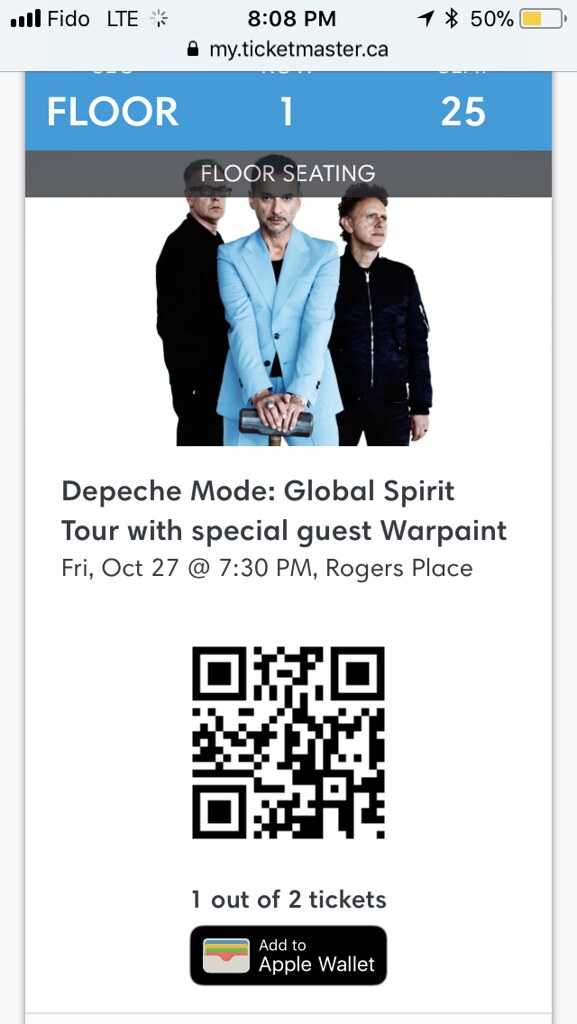This image is a full-color promotional piece displayed on a smartphone screen, primarily digital with an integrated photograph. At the top of the screen, there's a blue banner with white text, indicating the device status: 808 PM, LTE signal, and 50% battery charge. Below, the text announces details for the Depeche Mode Global Spirit Tour with special guest Warpaint, taking place on Friday, October 27th at 7:30 PM, at Rogers Place. The seating level is specified as Floor 125. The middle of the screen features a photograph of three men from Depeche Mode. Below the photograph, there's a QR code for one out of two tickets and an option to add the ticket to Apple Wallet. The colors in the image are vibrant, including baby blue, black, white, orange, yellow, and green, arranged in a vertical layout that moves from the device status at the top, down through the event details, photograph, and ticketing information.